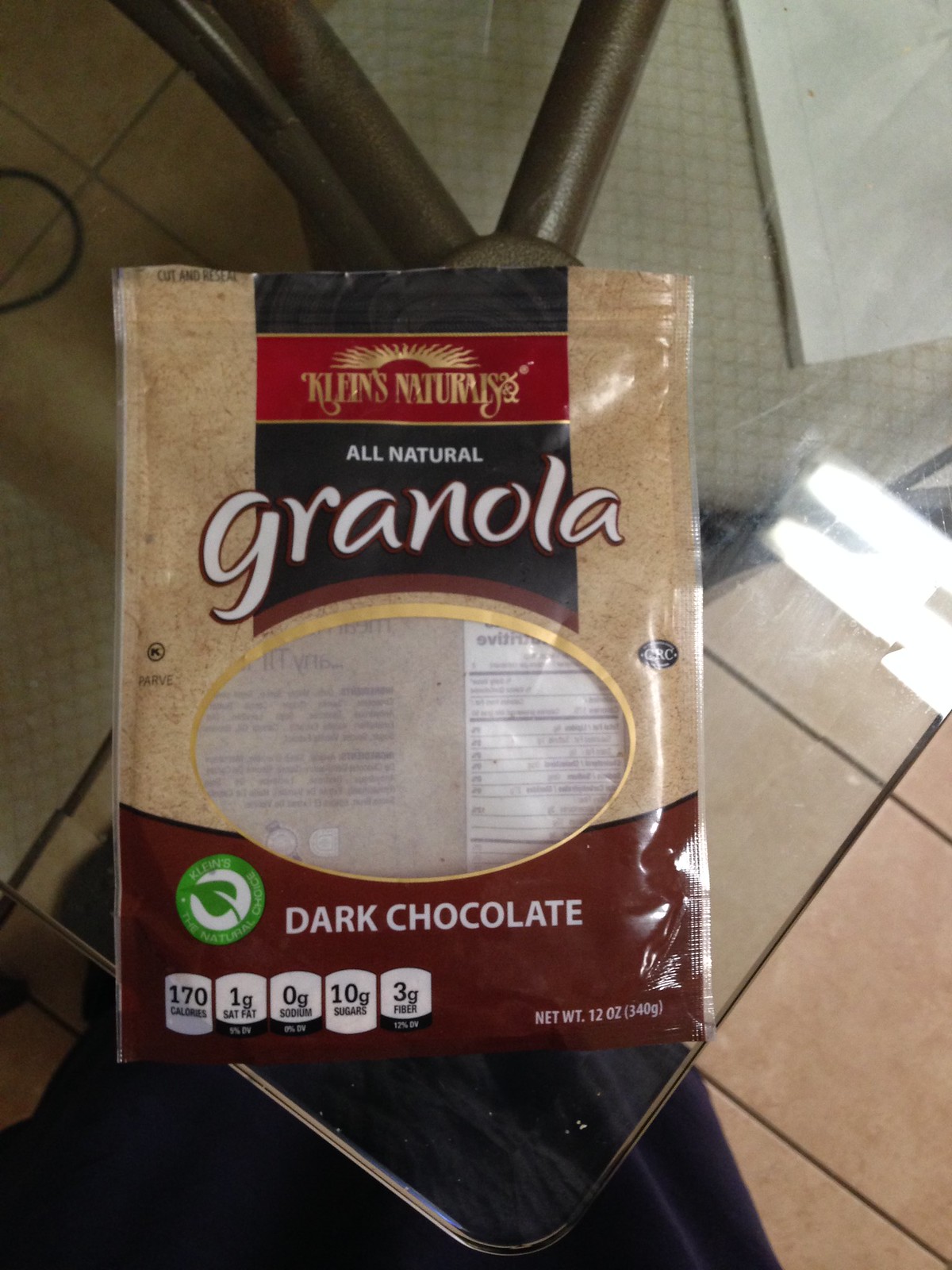This is a close-up color photograph of an empty granola bag that is placed on a clear glass tabletop, possibly plastic. The tabletop reveals light tan tiles underneath and features a shadowy dark metallic structure, which appears to be the table's legs. On the table, adjacent to the empty granola bag, there’s a sheet of white paper visible in the upper right-hand corner and a partially visible dark black object or image at the bottom of the glass surface. 

The granola bag itself is beige on the top and brown at the bottom, with a transparent plastic window through which the contents could be seen when it was full. A black strip at the top of the bag displays the brand name "Klein's Naturals" in gold writing enclosed in a narrow red frame, with "All Natural Granola" written in white text underneath. Below the window, it says "Dark Chocolate" in white. To the left of the window is a green and white round emblem, likely an organic or environmentally friendly logo, that reads "Klein's All Natural Choice." At the bottom left of the bag, there is nutritional information in black text on a white background, and on the bottom right, the net weight is indicated as 12 ounces. In the background, the light tan tile floor and a black fabric suggest the presence of a person nearby. Moreover, there is a round piece of a cord visible in the upper left-hand corner, adding a final touch to the intricate surroundings of the setting.